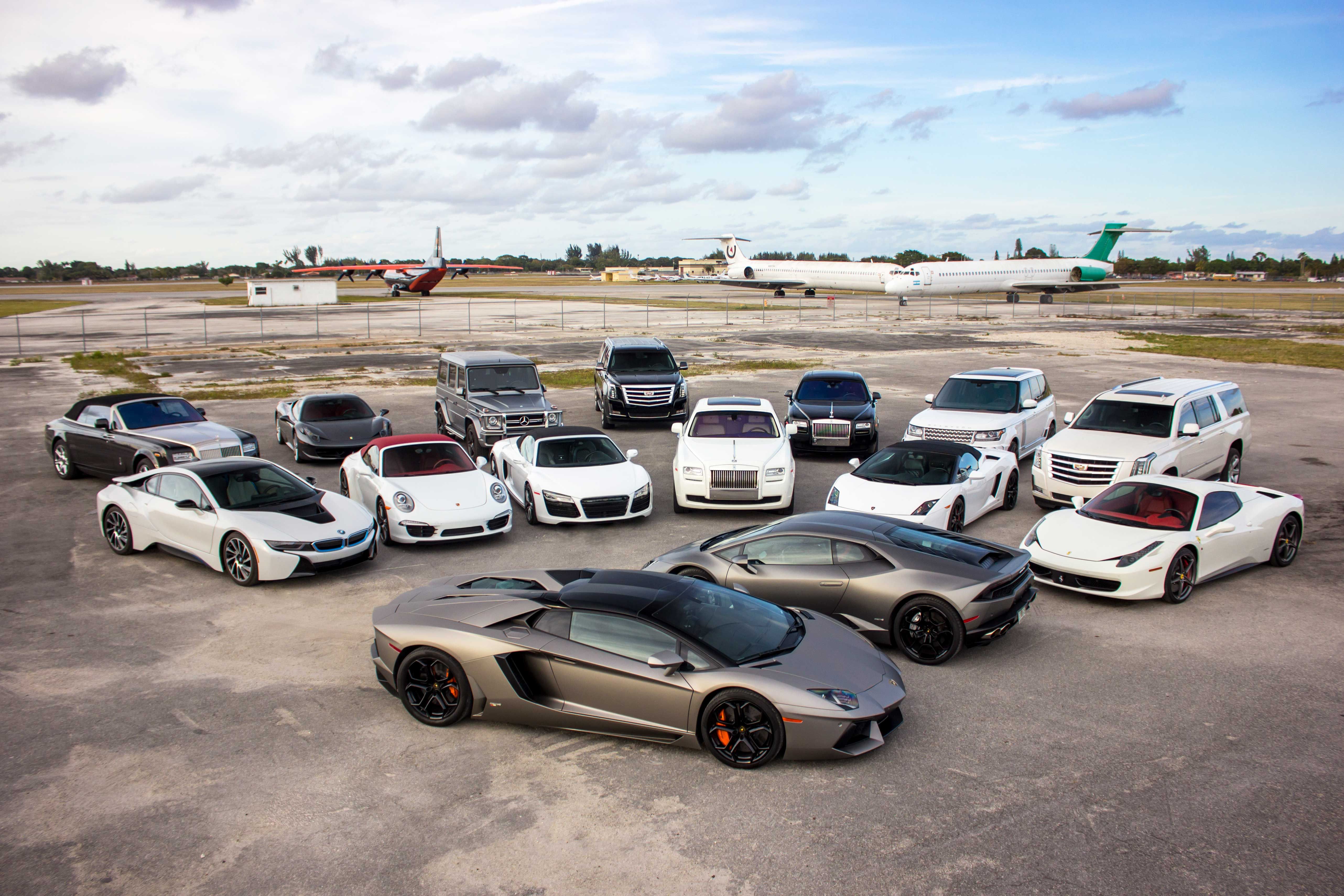This detailed photograph captures a striking scene of luxury and futuristic cars prominently displayed on an asphalt surface. The focal point of the image features 14 high-end sports cars, primarily in shades of white and dark silver, with a standout black vehicle and a van-like car adding variety to the lineup. The two most prominent vehicles in the front are sleek, dark silver sports cars, exuding a futuristic aesthetic.

As you move your gaze to the middle ground, you can see the cars arranged in a crescent shape, consisting of several white cars, predominantly from prestigious brands such as Mercedes, BMW, Porsche, Rolls Royce, Bentleys, Chevy, and Range Rover. The varied lineup suggests an exclusive collection of premium vehicles.

In the backdrop, at least three to four airplanes provide an interesting contrast to the ground vehicles. Two planes face each other, while another red-hued plane faces away from the camera. Additional planes include white aircraft with distinctive green and red markings. The sky above is a light blue, peppered with a considerable number of clouds, adding a dramatic overhead canopy.

Completing the landscape are distant trees and a view of the skyline, contributing to the open-air ambiance of this captivating scene. The attention to detail, from the arrangement of the cars to the positioning of the planes and the surrounding natural elements, makes this image a visually engaging composition.